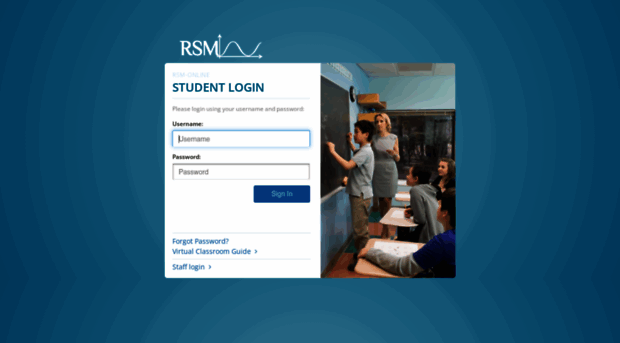The webpage features a gradient blue background that transitions from a lighter blue in the center to a darker blue at the edges. In the center, concentric rings of light blue radiate outward. At the top, the white text "RSM" is prominently displayed above a white chart depicting a wave with arrows pointing upward and to the right. Below this, the text "STUDENT LOGIN" appears in bold, blue, all-capitals letters. 

A gray subtitle urges users to "Please log in using your username and password." Beneath this instruction are two input boxes: the top box, outlined in blue and displaying a cursor icon, is labeled "Username," while the bottom box is for the password. Both boxes have placeholder text indicating their respective functions.

Directly below the password box is a blue "Sign In" button. Further down, a series of blue links offer additional options: "Forgot Password," "Virtual Classroom Guide," and "Staff Login."

On the right side of the page, an image depicts a classroom scene. Students are seated at desks, and a child is writing on a blackboard with chalk. The teacher, a woman in a gray dress, stands nearby. The classroom walls are painted blue, and a clock is mounted on an adjacent wall.